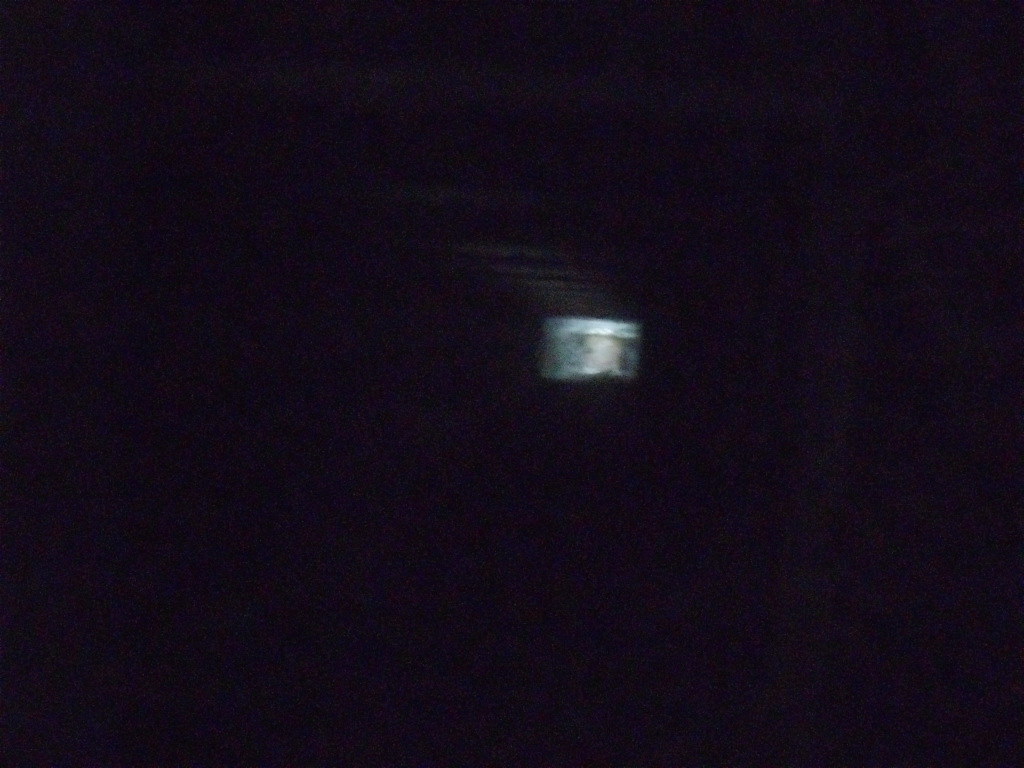The image features a predominantly dark, nearly black background, shrouded in a highly out-of-focus haze. At the center of this obscured backdrop lies a small, almost indistinguishable square. This square appears to have once been white, marked by its slight contrast against the surrounding dimness. Despite the poor focus, the square seemingly contains an element in its middle, hinting it could possibly be a screen or label. A white bar stretches horizontally across the top of the image, adding a subtle yet notable element of brightness to the somber composition. Overall, the scene is enveloped in darkness, with the central blurred square being the only discernible feature amidst the gloom.